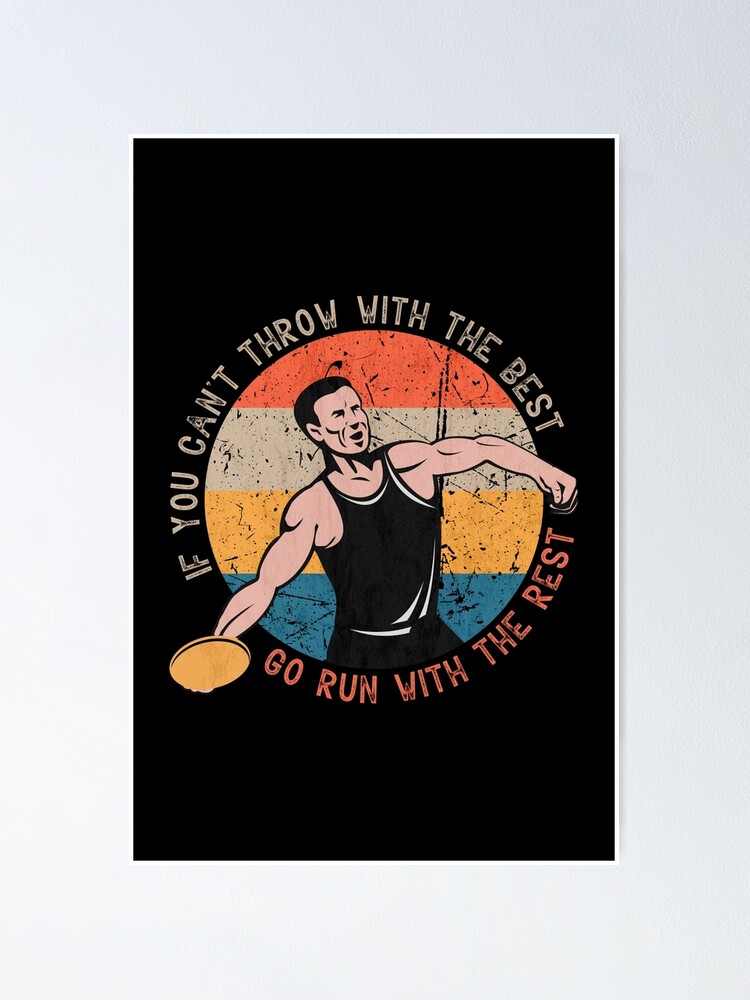The image depicts an animated, muscular man attempting a discus throw, set against a black background. He is clad in a sleeveless black tank top and black pants, highlighting his athletic build. The man grips a gold-colored discus in his right hand as he prepares to make the throw. Encasing him is a circle divided into segments of orange, off-white, yellow, and blue. Surrounding the circle, a white border features an inscription in two lines: "If you can't throw with the best, go run with the rest," with the top line in white text and the bottom line in orange.